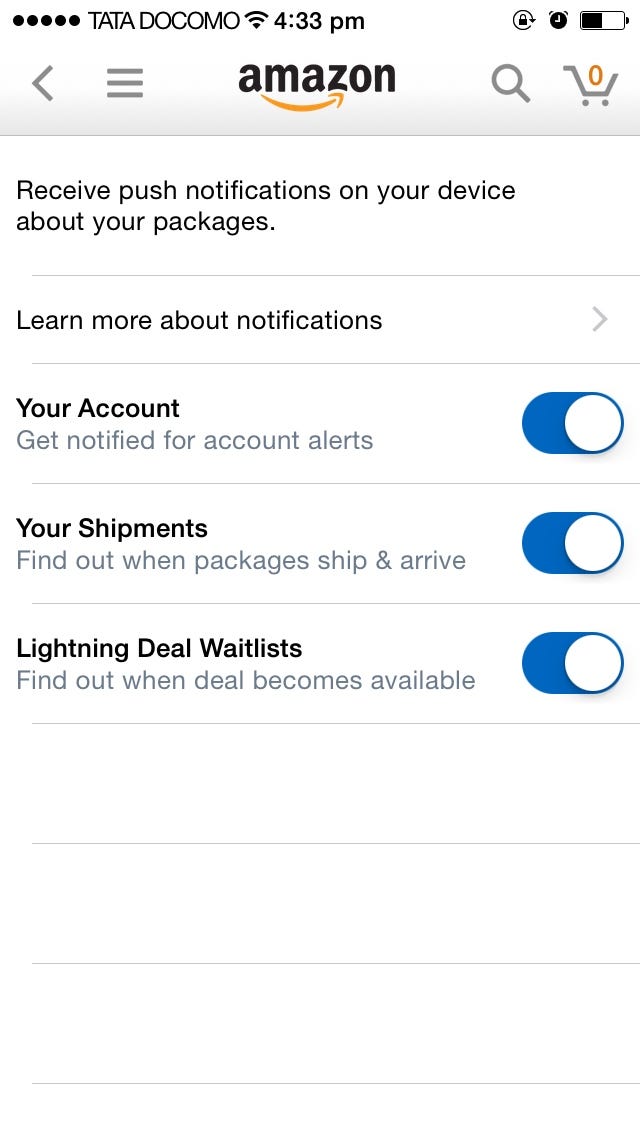This screenshot from a cellphone captures the settings page of the Amazon app. Positioned in the upper-left corner of the screen is the phone's toolbar displaying the carrier name "Pata Docomo," the time "4:33 PM," and a battery icon indicating approximately 40-45% charge. Dominating the top section of the app is the Amazon logo featuring the iconic "Amazon" text with the trademark smile beneath it. To the right of the logo is an empty shopping cart icon marked with a zero, and to the left, a back arrow.

The main section of the screen displays a white background with the text prompting users to "Receive push notifications on your device about your packages." Below this message is a link to "Learn more about notifications." Further down are toggle switches for different push notification options. The first option, "Your Account," is turned on and alerts the user about account-related notifications. The second option, "Your Shipments," is also activated, providing updates on package shipments and arrivals. The third toggle, "Lightning Deal Waitlist," is enabled to notify the user when new deals become available. This setup shows that the user has opted to receive all types of push notifications offered by the Amazon shopping app.